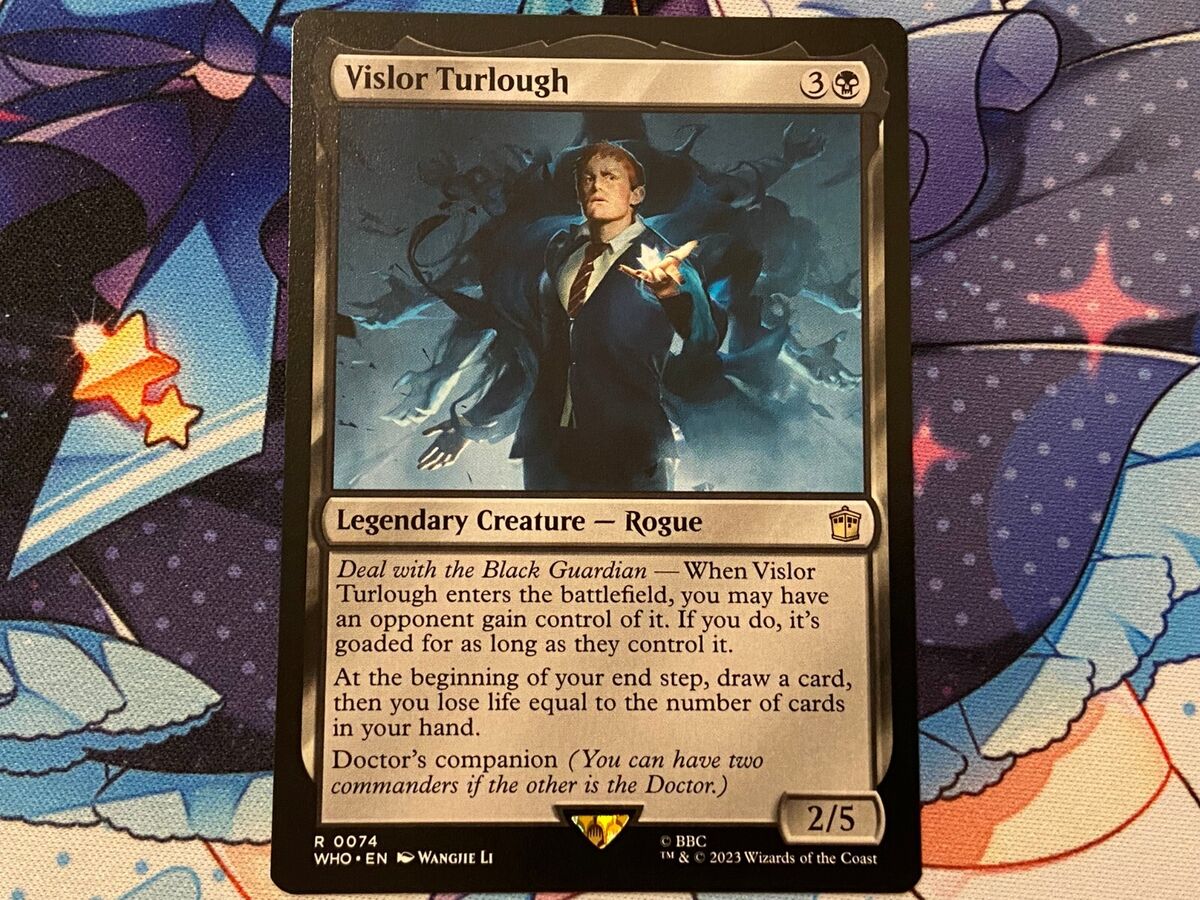This image depicts a detailed trading card named "Vizlor Turlow." The style is photographic, highlighting the gold card set against a black background. At the top, the card displays the name "Vizlor Turlow," a legendary creature classified as a rogue. The card features a white man in a dark suit, with a red tie, and white shirt. He is striking a dynamic pose with his hands spread apart, holding what appears to be a star in his left hand, while he gazes slightly upward. Surrounding him are grasping arms, adding a dramatic effect. The text reads: "Deal with the Black Guardian. When Vizlor Turlow enters the battlefield, you may have an opponent gain control of it. If you do, it's goaded for as long as they control it. At the beginning of your end step, draw a card, then you lose life equal to the number of cards in your hand. Doctor's Companion: You can have two commanders if the other is the doctor."

Beneath this text, the bottom right-hand corner displays the numbers "2/5," and in the bottom left-hand corner, there is "R0074." Additional details include the name "Wayne Wang" and affiliation markers "BBC, 2023, Wizards of the Coast." The aesthetic of the background is reminiscent of a Peter Max poster, featuring pop-up background stars, polka dots, curves, purple stars to the right, yellow stars to the left, and a pattern of blue, purple, and white polka dots underneath the card. This is further accentuated by green and blue clouds and orange elements in the bottom right-hand corner.